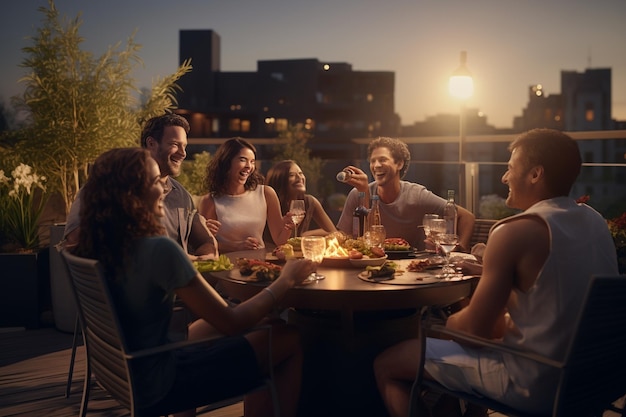The photograph captures a lively rooftop party featuring a group of six young adults, likely in their late 20s or early 30s, gathered around a circular table on an open terrace deck. The nighttime cityscape provides a stunning backdrop, illuminated by a nearby streetlight and a table centerpiece which reflects light, casting a warm, yellow glow over the scene. The friends, composed of both men and women, are all laughing and appear to be in the midst of a joyous conversation, indicating a delightful atmosphere. They are dressed comfortably in either sleeveless or short-sleeved tops, suggesting a warm evening. Each person holds a wine glass, and an assortment of cheese, fruit, and crackers is spread out on the table. A man in the center of the group is holding a cane adorned with an elaborate top. The setting is further enhanced by the presence of potted plants and a taller green tree to the left, contributing to the relaxed and inviting ambiance of this cheerful gathering.